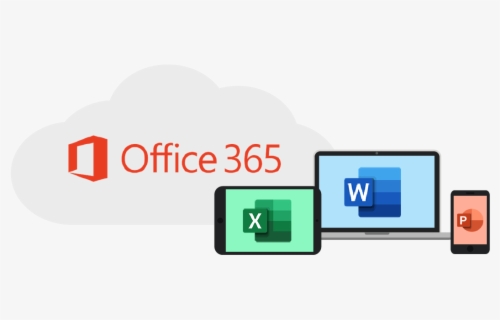The image is a detailed screenshot showcasing the Office 365 logo against a grey background. On the left side of the image, there is a light grey cloud with subtle, almost 3D edges, which might have been mistaken for screen marks initially. 

The prominent Office 365 logo is featured in red, with a distinctive doorway-like symbol on its left. To the right of the logo, the image presents a series of infographics that represent different devices: a tablet, a laptop, and a mobile phone.

The tablet is depicted in landscape mode with noticeable bezels at the top and bottom. It displays an Excel spreadsheet, characterized by a green background and a white "X."

Next, the laptop image shows a device with a grey base and a black trim surrounding the screen. The display features the Word application icon, set against a background of four blue gradients and a lighter blue backdrop.

The mobile phone illustration features substantial bezels at the top and bottom, with black edges. The screen shows an icon for PowerPoint, marked by a white "P" on a peachy orange background with a small orange square. To the right of these infographics, there's a circle partially colored in a lighter orange, with the rest in a darker orange, further reinforcing the association with PowerPoint.

In summary, this image serves as a comprehensive visual representation of the Office 365 suite and its compatibility with various devices, highlighting Excel, Word, and PowerPoint applications.